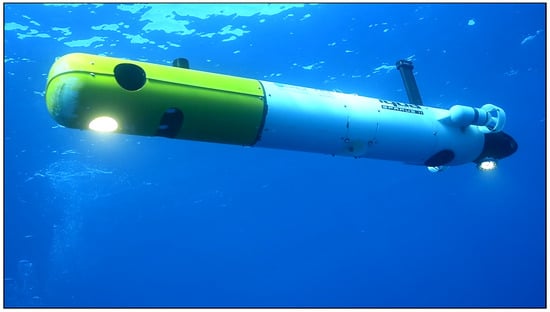This underwater photograph captures a detailed view of a small submersible facing upwards, with the camera positioned below, looking towards the ocean's sunlit surface. The submersible, elongated and cylindrical, features a mix of color: predominantly white with a yellow section about a third from the front. The rear of the vessel tapers into a black cone shape. The image highlights various details, including multiple lights—one bright round light at the front, one attached to the rear cone, and another nearby. The submersible also sports two small white propellers jutting from the fuselage's sides. Additional features include a prominent porthole within the yellow segment and a black periscope extending from the rear. The sunlight filtering through the water on the left adds a striking contrast to the deep blue ocean encasing the submersible.